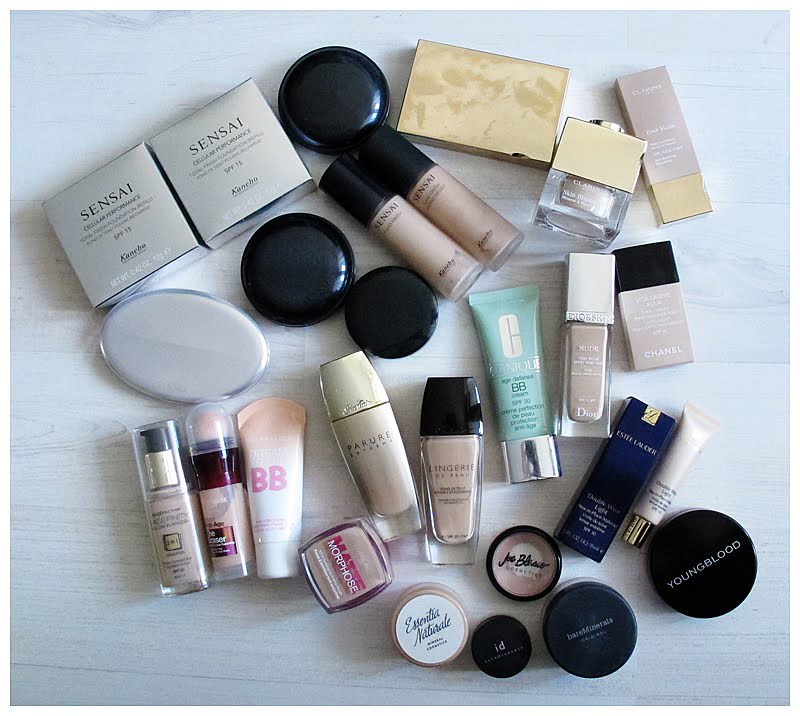This photograph showcases an assortment of makeup products meticulously arranged on a white wooden surface, accentuated with subtle gray wood grain. 

In the upper left corner, there are two silver boxes with the brand name "Sensai" elegantly printed in black font. Below "Sensai," there's smaller, illegible black text. To the right of these boxes, a sleek black compact is positioned.

Further to the right, there is a sophisticated golden square box, followed by a small, square glass ampoule labeled "Clairol," adorned with a golden, screw-off lid. Next to the ampoule, a cream and gold rectangular box with white writing stands prominently.

Descending to the next row, two small glass containers come into view. These rectangular containers, with rounded edges and black lids, also display the "Sensai" branding. Below them, two round black compacts and an oval white compact are neatly aligned.

In the bottommost row, two lipsticks housed in elegant little glass containers complete the array, exemplifying a diverse and well-organized collection of beauty essentials.